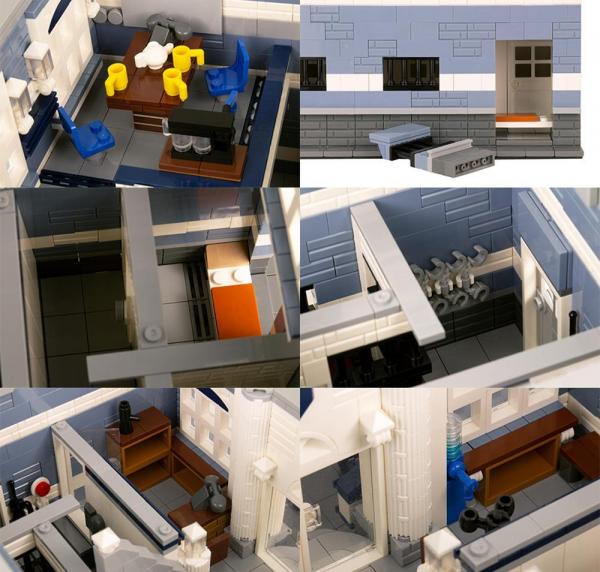This image is a detailed collage of six Lego-built dioramas, each segment of equal size, illustrating different aspects of what appears to be a Lego jail or police station. The top left image showcases an office-like room with Lego chairs, a brown Lego table adorned with yellow Lego coffee cups, a gray Lego telephone, and a black Lego coffee pot, possibly an interrogation or break room. The top right image displays the light blue and gray exterior of the building, indicating broken blocks scattered at the top right corner. The middle left segment reveals a small jail cell containing an orange bed. Next to it, the middle right image depicts part of a jail hallway, complete with handcuffs hanging on the wall. The bottom left captures another office space with a desk and a telephone, while the bottom right provides an additional angle of this reception or office area. The Lego construction is illuminated with good lighting, emphasizing its sturdiness and the smooth, properly arranged pieces. The colors featured prominently include grays, browns, oranges, and blues, underscoring the realistic and intricate design of the miniature setup.